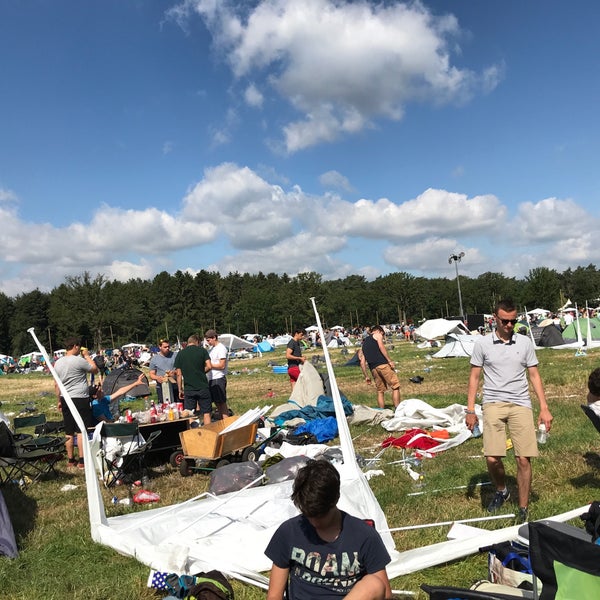This outdoor photograph captures a busy, vibrant scene unfolding under a blue sky dotted with fluffy white clouds. Below the sky, a dense line of tall green trees stretches across the background, framing a lively camping or event area. Scattered throughout the grassy field are numerous white canopies and assorted tents in hues of blue and red. In the foreground, a person in a black shirt with the word "Roman" emblazoned on it is setting up a white canopy that currently rests on the ground. To the left, a table is set up with condiments and bottles, suggesting a meal area where several people, mostly in shorts and t-shirts, are gathered. The left side of the image features a mix of individuals: one in a gray shirt and black shorts, and another in a blue shirt with a black hat. A prominent group stands nearby, including a person with sunglasses on their head sporting a blue shirt and dark pants, and another individual in a gray hat, white shirt, and black pants. The scene is lively yet somewhat cluttered, with visible debris and plastic bags tied up, indicating ongoing setup or takedown activities. Overall, the photograph offers a detailed snapshot of the communal effort and casual atmosphere of this outdoor event or camp.